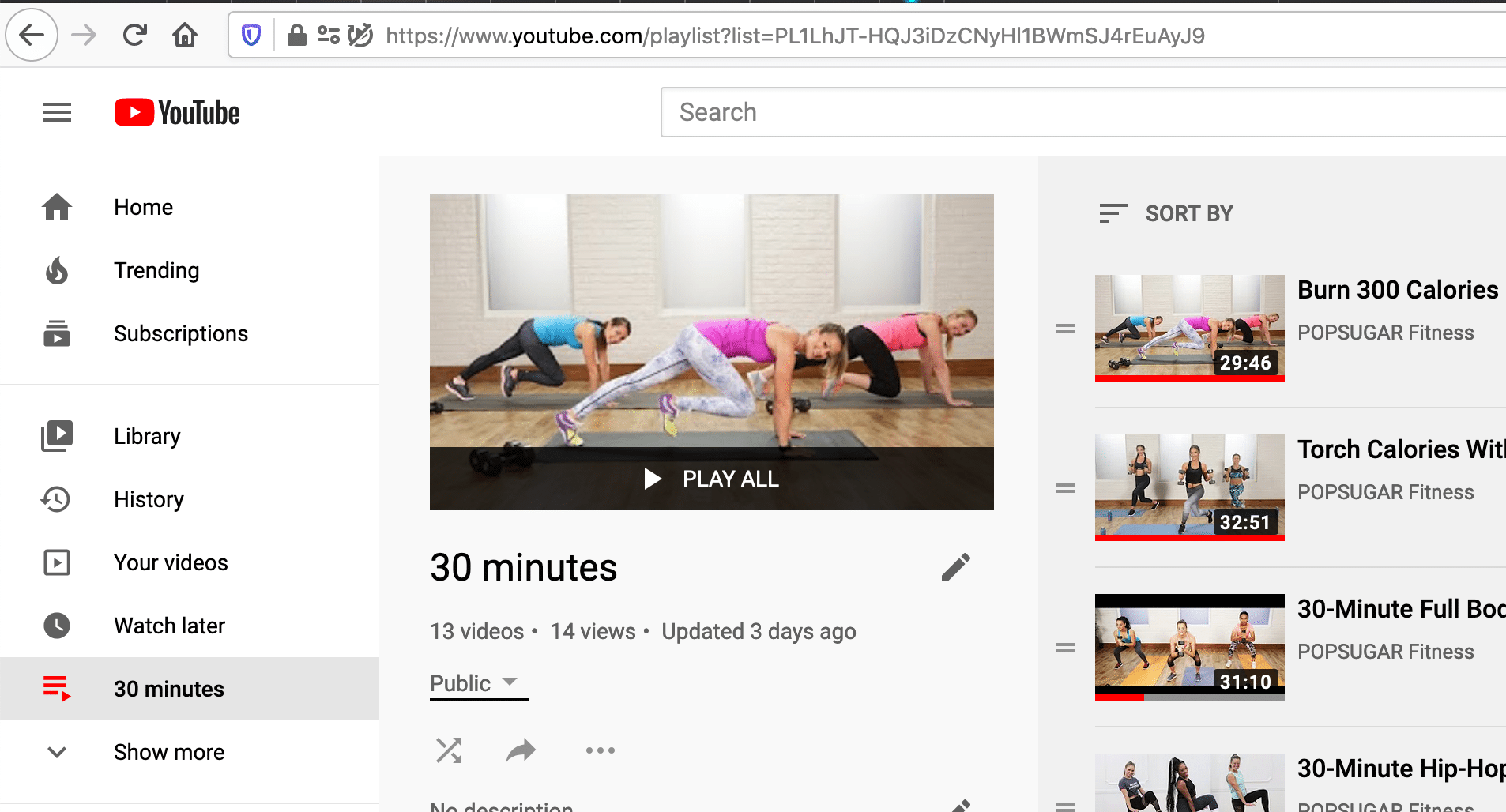This image features the desktop version of the website YouTube. At the top of the page, the address bar displays the YouTube URL with a focus on a playlist section. The webpage itself is displayed with a white background, indicating that the user is not utilizing the dark mode.

In the top left corner, the image shows the navigation drawer icon, followed by the iconic red and white YouTube play button, with the word "YouTube" written in black next to it. To the right of this logo, there is a prominently placed search bar.

On the left side of the page, a vertical list of navigation tabs is visible, including options such as Home, Trending, Subscriptions, Library, History, Your Videos, and Watch Later. Among these, the "Watch Later" section is highlighted with a light gray box and a red icon next to it, indicating it is the currently selected tab.

Beneath these navigation tabs, there is an option to "Show more." On the right side of the page, under the "Watch Later" section, there is a list of videos. A notable entry in this list is a playlist labeled "30 minutes" which features a thumbnail of three women exercising. This playlist is noted to contain 13 videos.